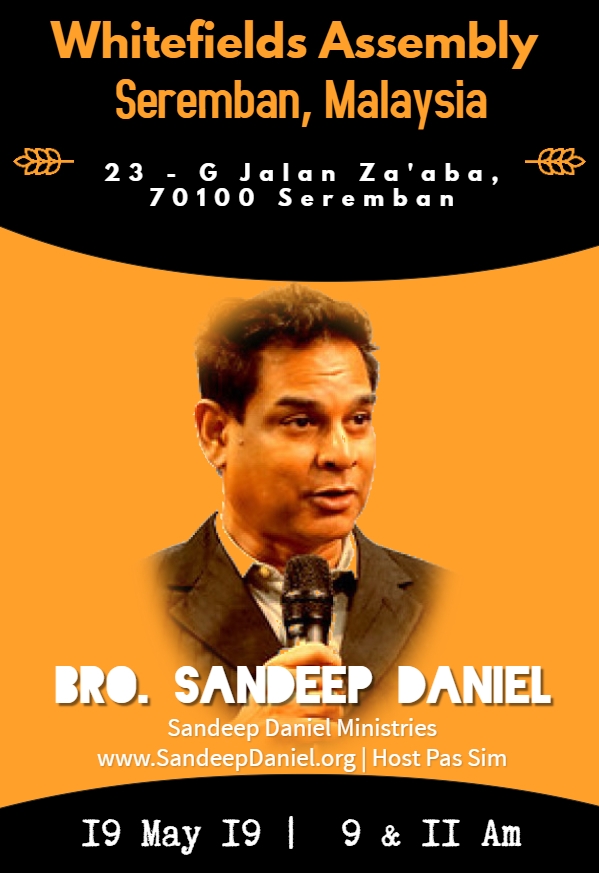This is a detailed advertisement poster for a religious event hosted by Whitefields Assembly in Seremban, Malaysia. At the top of the advertisement, presented in orange letters, it says "Whitefields Assembly." Below this, in white letters, the location is detailed as "23-G Jalan Zaaba, 70100 Seremban, Malaysia." Featuring prominently in the center is a photograph of Brother Sandeep Daniel from Sandeep Daniel Ministries. Brother Sandeep Daniel appears to be of Indian descent, possibly in his 40s or 50s, dressed in a tan button-down collared shirt with a black blazer, and holding a black microphone. His name is highlighted in white letters below the image while the URL for his ministry, "www.sandeepdaniel.org," is also provided. The poster specifies the event date and times as "19 May" with sessions at "9 and 11 a.m." The background of the poster is predominantly orange, framed by circular bands of black at the top and bottom, adding visual contrast to the design.